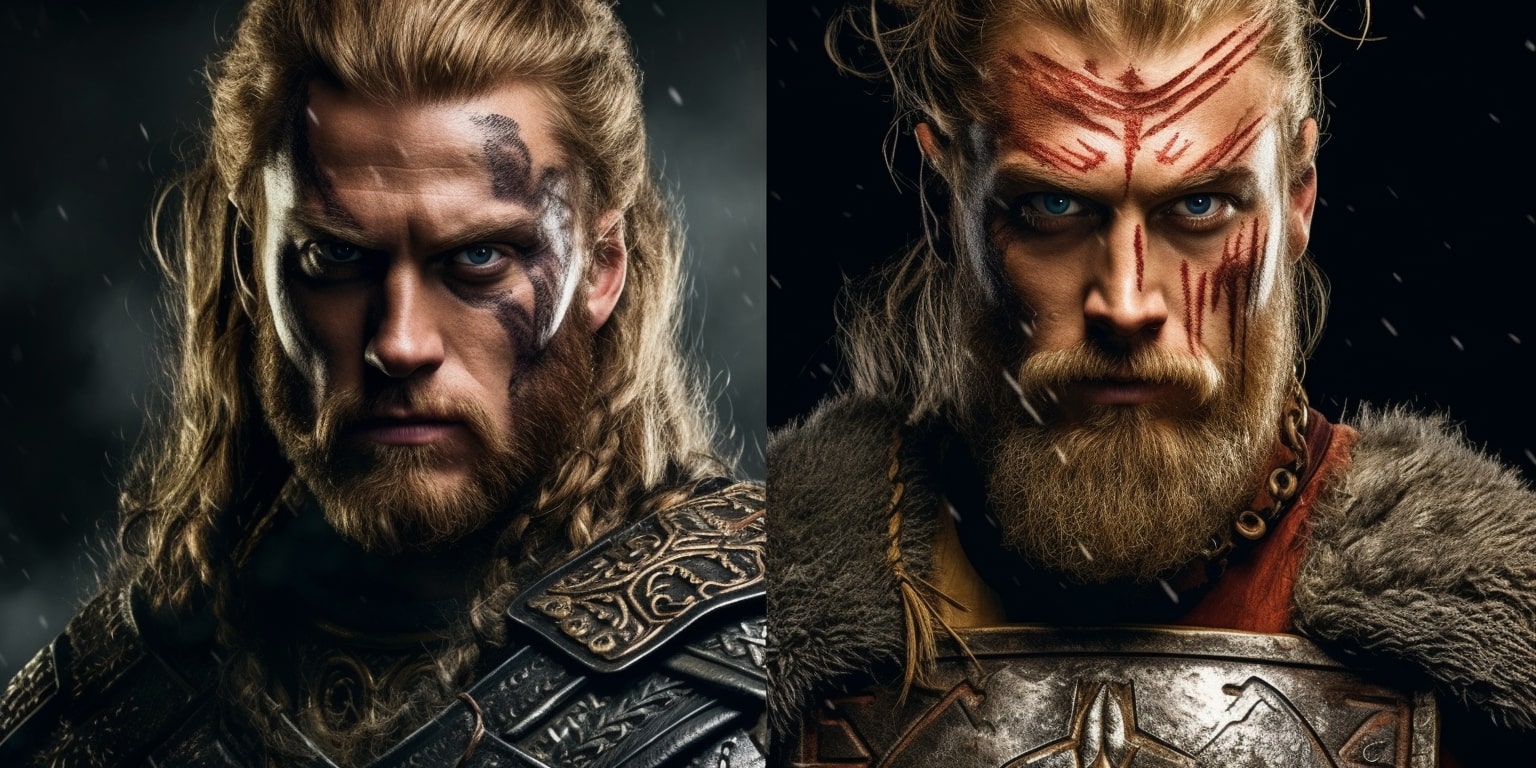This image features two digital renderings of the same man, possibly from a video game or a book, set in a medieval or fantasy world. On the left, he appears with fair skin, light brown hair, and a beard, emanating a very serious expression. His long hair flows freely, and his face is adorned with dark marks or tattoos. He is dressed in ornate black and gold armor, suggestive of a knight or a high-ranking warrior. On the right, the same man appears aged, with longer hair pulled back and a longer beard. His face is strikingly marked with red paint or blood, featuring a bird motif and lines that heighten his fierce appearance. His attire consists of a rugged metal chest plate and a fur collar, evoking the look of a barbarian. The fur on his shoulders resembles that of a wild animal, like a wolf, contributing to his formidable and violent presence.